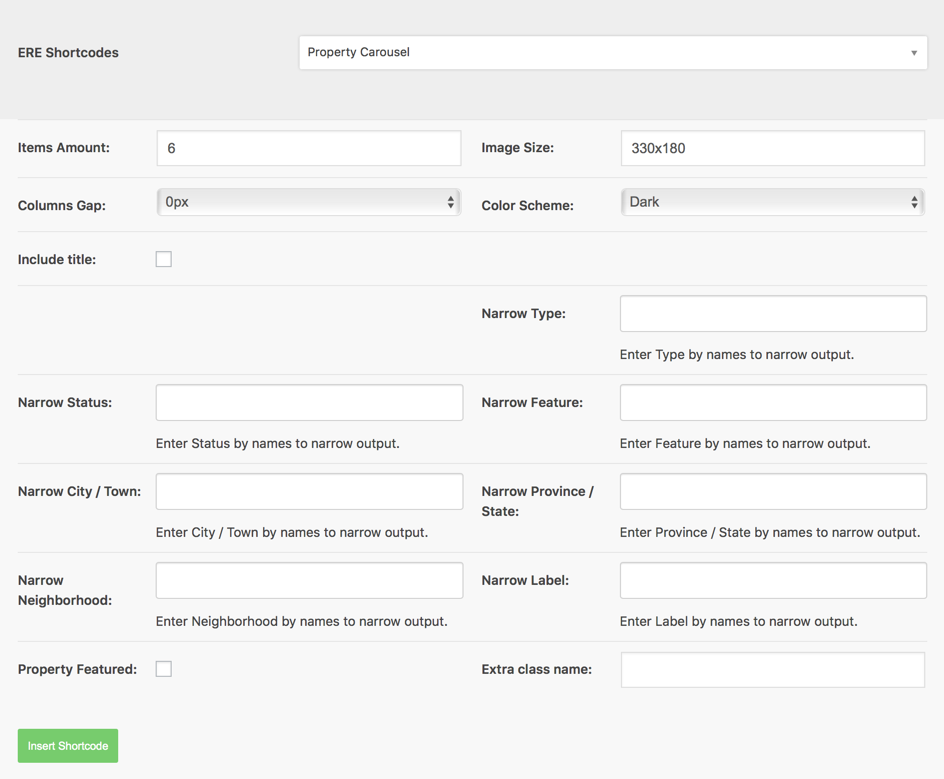This image is a screenshot from an unspecified website displaying the configuration options for ERE shortcodes pertaining to a property carousel. The interface is divided into various sections, each containing different parameters. At the top, it specifies that the property carousel will display 6 items with an image size of 330 x 180 pixels and no column gap, utilizing a dark color scheme. Several filters are available, such as title, type, status, feature, city/town, province/state, neighborhood, and label, each requiring specific inputs to narrow the output. It is noted that the 'Include title' and 'Property feature' checkboxes are not selected. Below these options, there is an input field labeled 'Extra ClassName' for additional styling. The bottom-left corner of the interface features a green rectangular button with white text that reads "Insert Short Code." The image is strictly textual and lacks any photographic or illustrative elements, as well as any people, animals, plants, buildings, or vehicles.